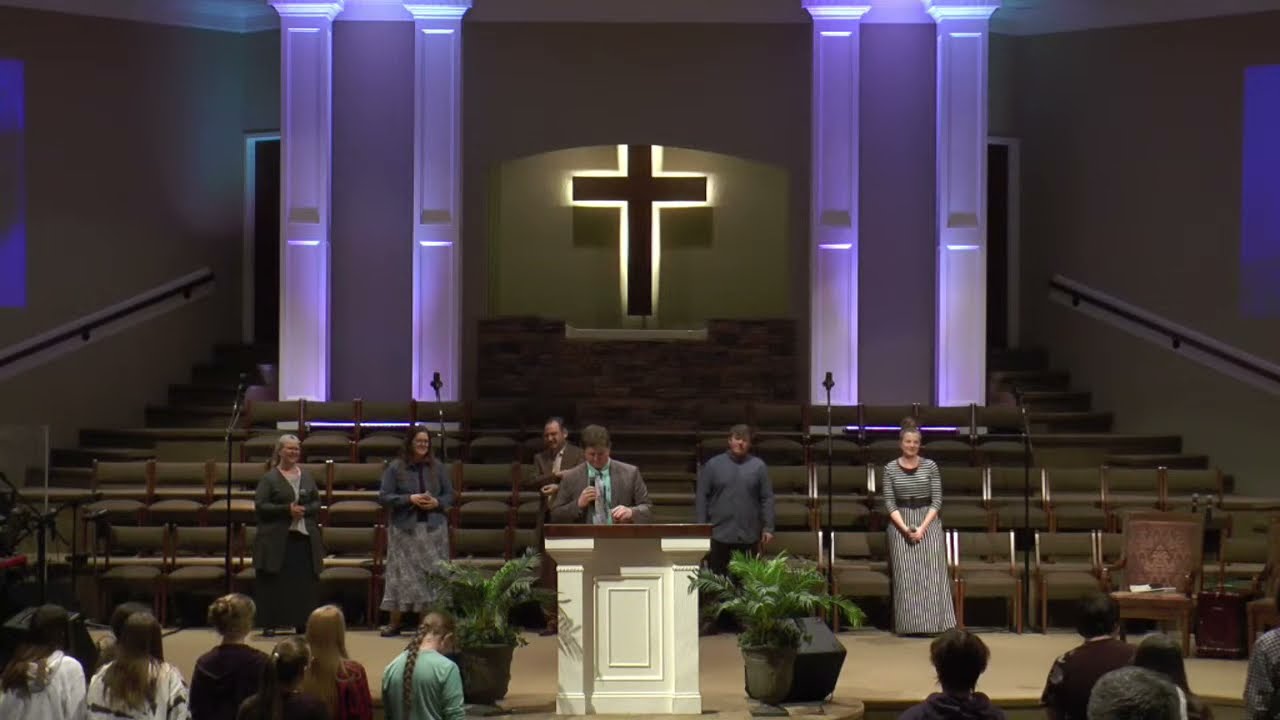The image captures a lively worship service within a spacious church. At the forefront, a Caucasian gentleman with brown hair, dressed in a gray suit and teal collared shirt, stands behind a prominent white pulpit, holding a microphone. The pulpit features two white pillars and a rectangular frame design. Flanking the pulpit are large green ferns, adding a touch of nature to the scene. 

Five individuals—two women to the speaker's left, two men directly behind him, and another woman to his right—stand supportive on the stage. Beyond them, a congregation, seemingly engaged and attentive, stands facing the speaker, suggesting a significant moment in the service.

The backdrop is striking, with a large, luminescent wooden cross at the center of the back wall, glowing with a yellowish-white light. On either side of the cross are pairs of white pillars, each glowing with a purple hue, and beside them are assumed exit doors. Handrails extend along the left and right walls, guiding viewers down the steps that meet several rows of chairs positioned between the pillars, filling the room from wall to wall. This vivid setting is delivered from an overhead perspective, showcasing the structural and atmospheric elements of the church.